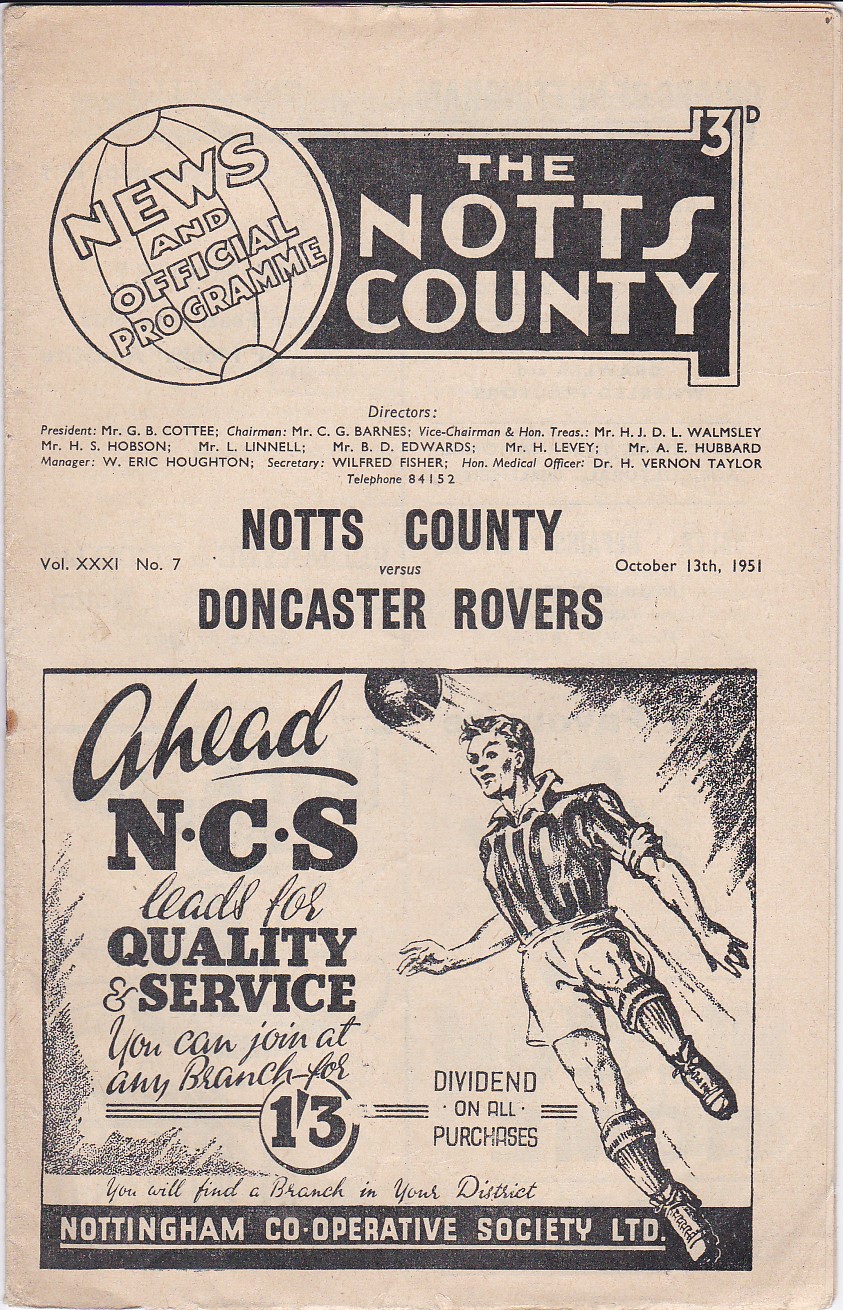This image depicts an aged, yellowing newspaper or magazine page, predominantly in black and white, though the paper's yellowing gives it a tan hue. The top of the page features a black box with the heading, "Knott's County," accompanied by a small "3D" in the top right corner. Beneath this, a circular globe design contains the text "News and Official Program." Below this, the directors of Knott's County are listed, followed by the event headline "Knott's County versus Doncaster Rovers." The issue information indicates it is Volume XXXI, Number 7, dated October 13, 1951. A detailed illustration shows a male European soccer player with short hair, wearing a white t-shirt bearing the letters "NCS," along with white shorts and socks. The player appears to be heading a ball. To the left of this image, text reads, "Ahead, NCS leads for quality service. You can join at any branch for $1.33 dividend on all purchases. You will find a branch in your district." The document ends with the "Nottingham Co-operative Society Ltd.”